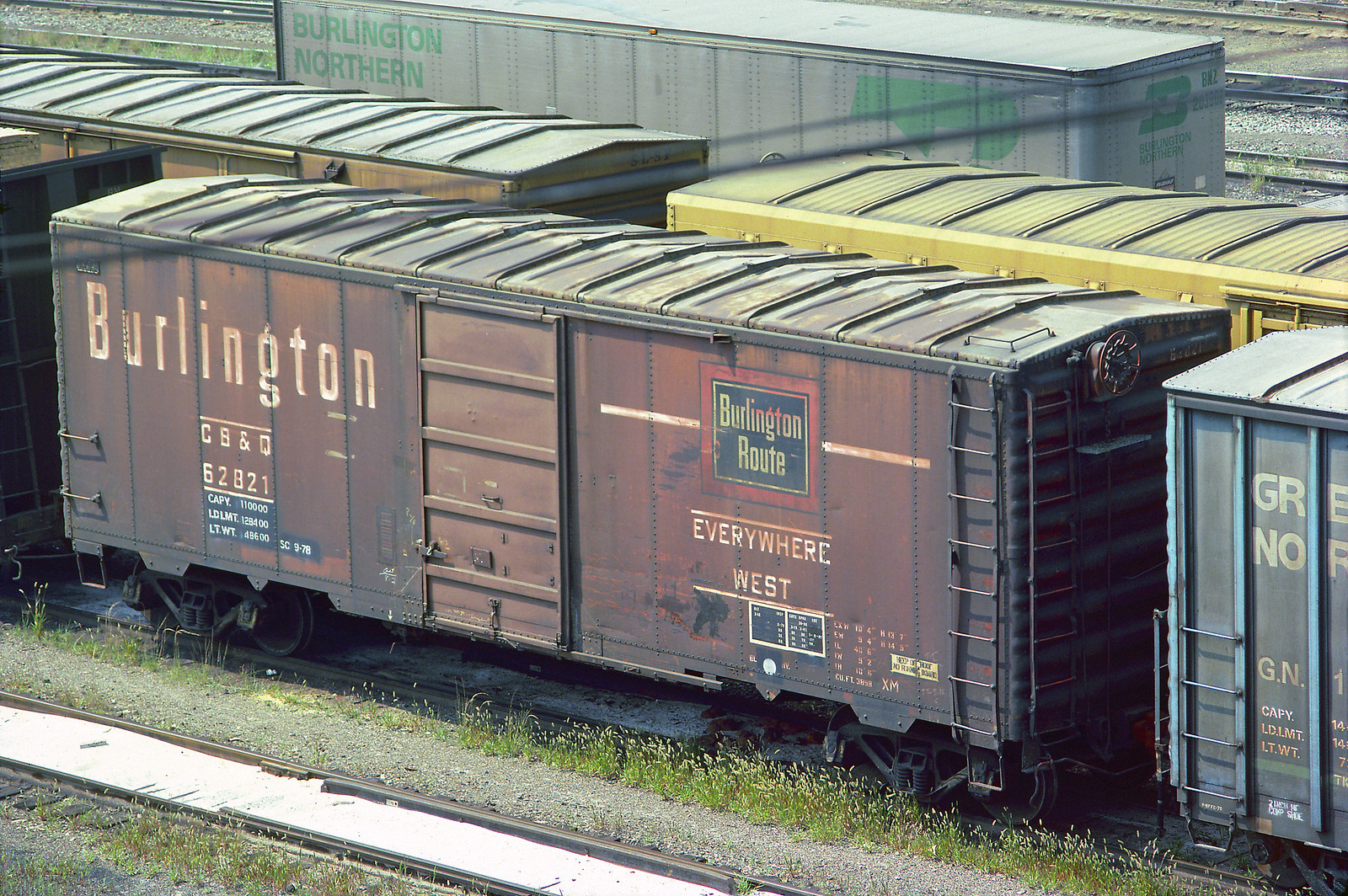The image depicts a bustling train yard with a collection of railroad cars positioned both side-by-side and end-to-end, creating a landscape that resembles an old, possibly abandoned, junkyard. The central focus is on a brownish-orange Burlington train car, prominently featuring the "Burlington Route" logo within a red rectangular border and slogan "Everywhere West." This car is detailed with the markings "CB&Q 62B21," "CAPY 110000," and "LD LMT 128400." Surrounding this central car are at least six other train cars, including a distant yellow car and a gray car identifiable as part of the Burlington Northern line. The tracks they rest upon are lined with high weeds with white tips and patches of gravel, suggesting a lack of recent maintenance. The metal surfaces of the cars exhibit rust, indicating age and wear. Additional tracks can be seen in the background, unoccupied by any train cars. The overall scene conveys a sense of inactivity, with the train cars seemingly waiting in limbo for their next journey.